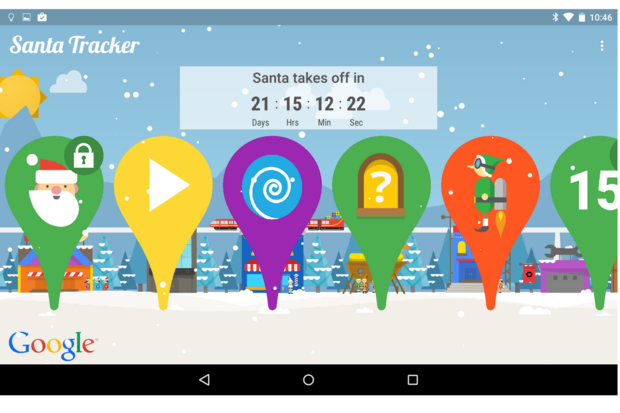The image is a rectangular screenshot with a dark blue background at the top, featuring several icons. In the top-left corner, there are some unidentified icons, while the top-right corner displays a Bluetooth icon, a Wi-Fi icon, a battery indicator showing more than 50% charge, and the time, 10:46.

Below this section is a picture that shows a blue sky with snowflakes falling, represented by white dots. On the left side of the picture, the text "Santa Tracker" is displayed. In the center, it reads: "Santa takes off in 21 days, 15 hours, 22 minutes and 12 seconds." Beneath this, there are several map pins similar to those on Google Maps:

1. A green pin with an image of Santa Claus and a lock.
2. A yellow pin with a white play button.
3. A purple pin with a blue circle and white swirls inside.
4. A green pin with a brown window, yellow interior, and a white question mark.
5. A red pin featuring an elf facing left, equipped with a jet pack.
6. Another green pin with the number 15 in the bottom-left corner.

At the bottom, there's a black section containing navigation buttons: a left-pointing triangle on the left, a circle in the middle, and a square on the right. The Google logo can also be seen on the green pin with the number 15.